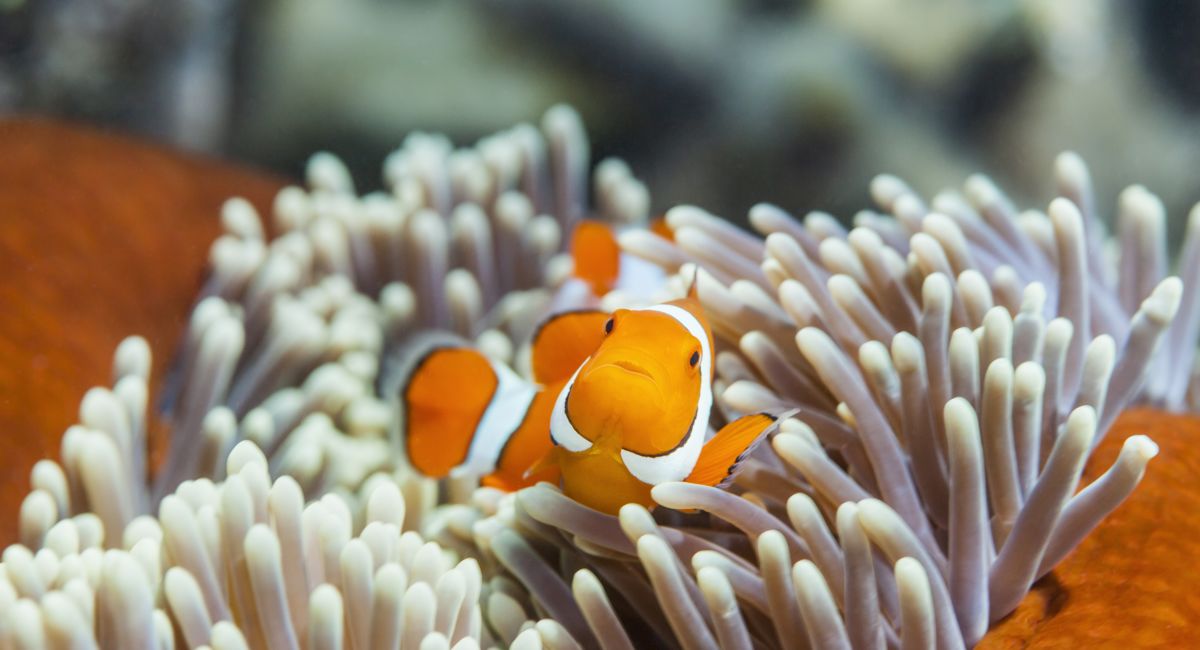This vivid underwater photograph captures a charming clownfish nestled at the bottom of the ocean amidst a thriving coral reef. The clownfish, with its striking orange body adorned with iconic white stripes outlined in black, is centrally positioned in the image, gazing slightly upwards. Its small, black eyes add to its endearing appearance. Surrounding the clownfish are creamy white and brown sea anemone tentacles that echo the hues of the reef. On either side of the anemone, there are bright orange rocks, adding to the vibrant color palette of the scene. The blurred background of the photograph showcases a mottled mix of black, tan, and gray tones, enhancing the focus on the vividly colored clownfish against the peaceful marine backdrop. This photo, reminiscent of a scene from "Finding Nemo," is a captivating snapshot likely taken by a marine biologist or an underwater diver, and it beautifully highlights the serene and vivid underwater world.